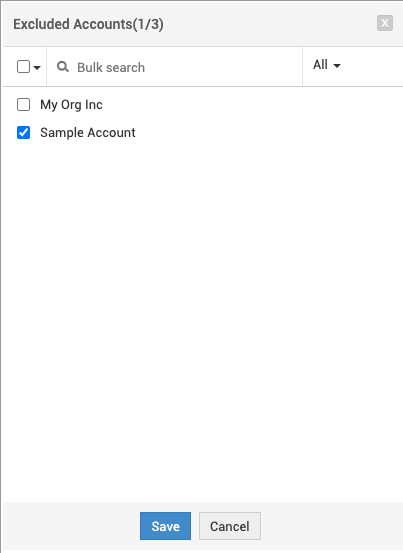The image displays a screenshot of the settings interface from an application. The interface features a clean design with a white background and grey borders at the top and bottom. At the top of the window, there is a label that reads "Excluded Accounts [1/3]", indicating a settings section related to account management. Adjacent to this label on the right is a close button, identifiable by a cross icon, which users can click to exit the settings window.

Below the header, there is a search utility labeled "Bulk Search" accompanied by a magnifying glass icon, suggesting a functionality to search through multiple items. To the right of the search bar is a checkbox with a downward arrow, symbolizing a dropdown menu or selectable options. This checkbox is turned on, revealing two options beneath it— "My Org Inc" which is unchecked, and "Sample Account" which is checked, indicated by a blue tick.

On the right-hand side within the header bar, there is an "All" button with a downward selection arrow, providing a broader filtering or selection capability. At the bottom of the settings window, there are two buttons: "Save" and "Cancel." The "Save" button is highlighted in blue with white text, indicating it's the action button, while the "Cancel" button is in grey with black text, offering an option to discard changes.

This interface allows users to manage account exclusions by selecting the desired settings and saving their preferences with the provided buttons.